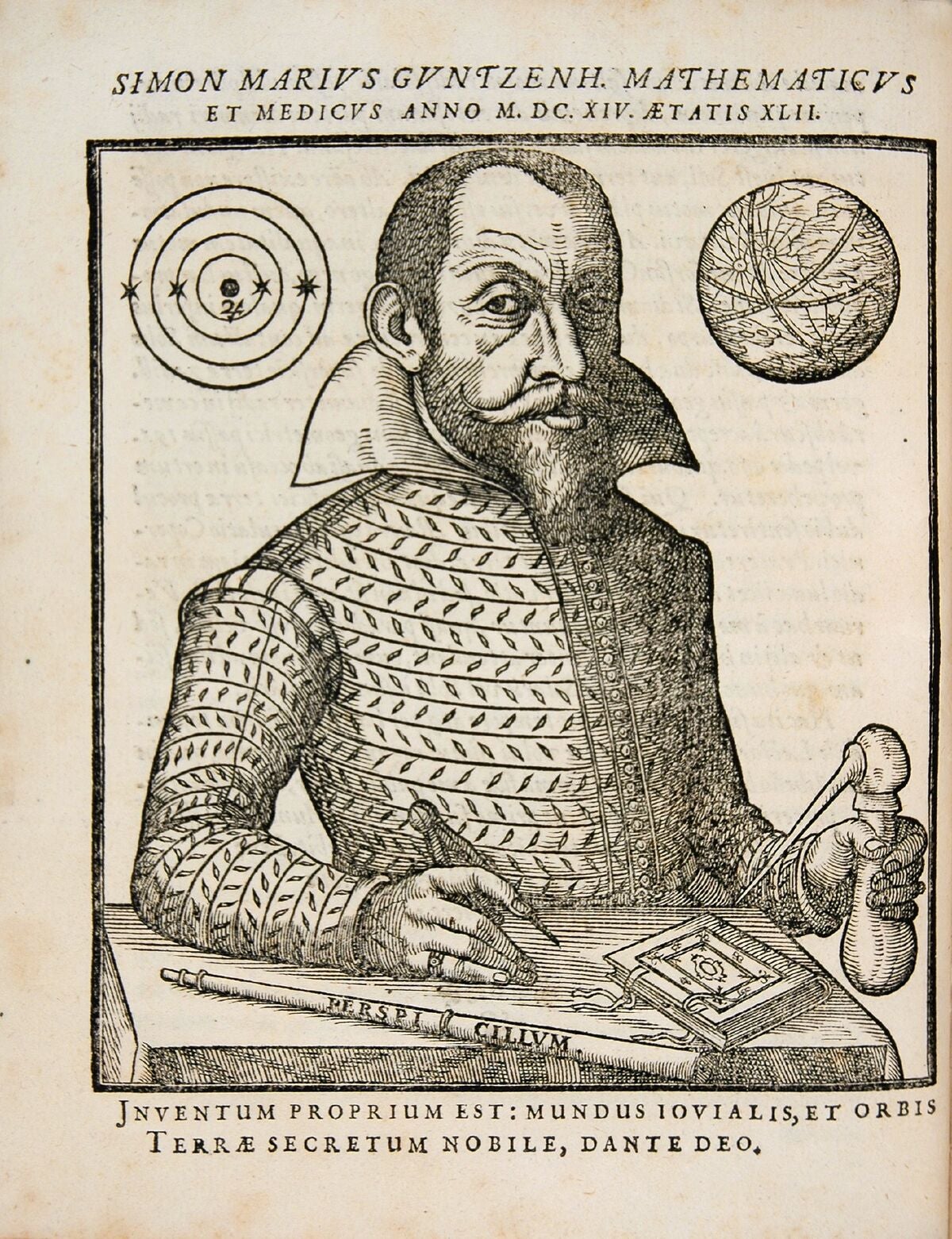The page from the book features a highly detailed, old-fashioned illustration, likely from an ancient text, drawn in a traditional crosshatch style with black ink on white paper. At the center of the image, a man with a long beard and a handlebar mustache is depicted wearing a form-fitting, formal tunic with a large, curled-up collar. In his hands, he holds various scientific instruments, including a tweezer or possibly fine compass, and a small squirt bottle or protractor, suggesting he might be a scientist or a mathematician engaged in experiments.

To the left of the man's head is a diagram representing the planetary solar system, while to the right is an illustration of a globe. Additionally, in front of him lies a flute, beside which is an open book. Above and below the central image, printed in black text, are various letters and words, including "S-I-M-O-N M-A-R-I-V-S, G-V-N-T-Z-E-N-H, M-A-T-H-E-M-A-T-I-C-V-S, E-T-M-E-D-I-C-V-S," hinting at the man's identity, possibly Simon Marius, and potentially suggesting his dual roles in mathematics and medicine. The text also includes a date formatted as Anno MDCXIV8, further emphasizing the historical context of the illustration.